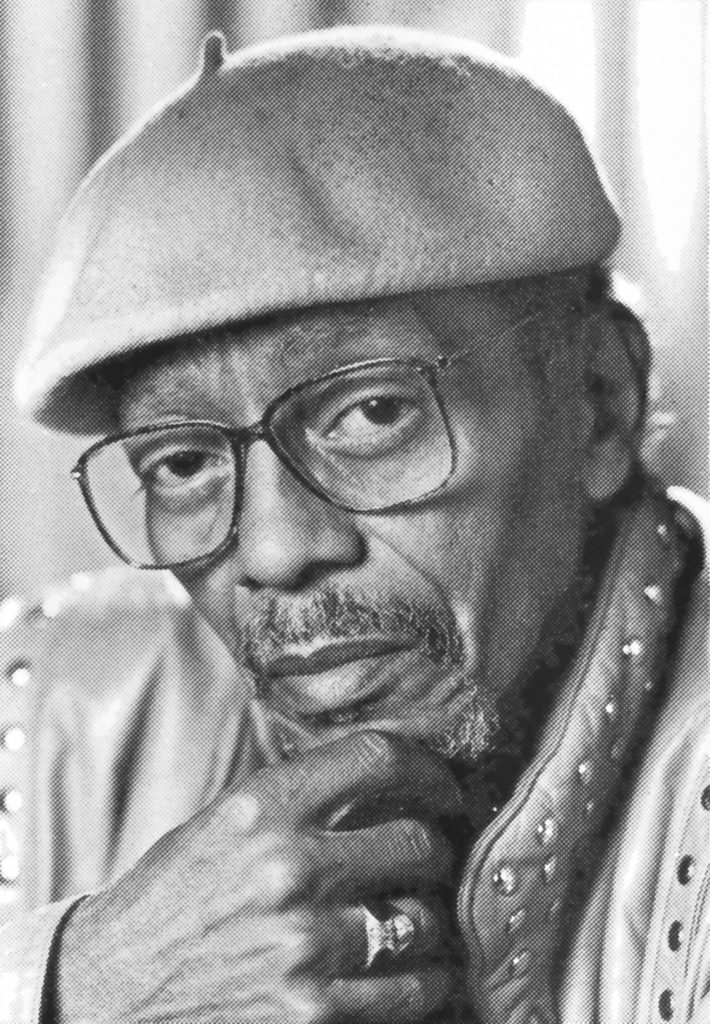The image portrays an African-American man, likely in his mid to late 60s, sitting with his right hand thoughtfully propped on his chin, giving him an inquisitive and intellectual demeanor. He wears a dark-colored jacket adorned with gold studs and a shiny gold ring on his finger, adding a touch of elegance to his appearance. His attire includes a small French beret, and he sports glasses, a mustache, and a beard. His expression is serious and somewhat uninviting, with eyes that seem to question or challenge the observer. The photograph, rendered in monochromatic shades of black, white, and gray, centers the man directly in the frame, highlighting his contemplative pose.